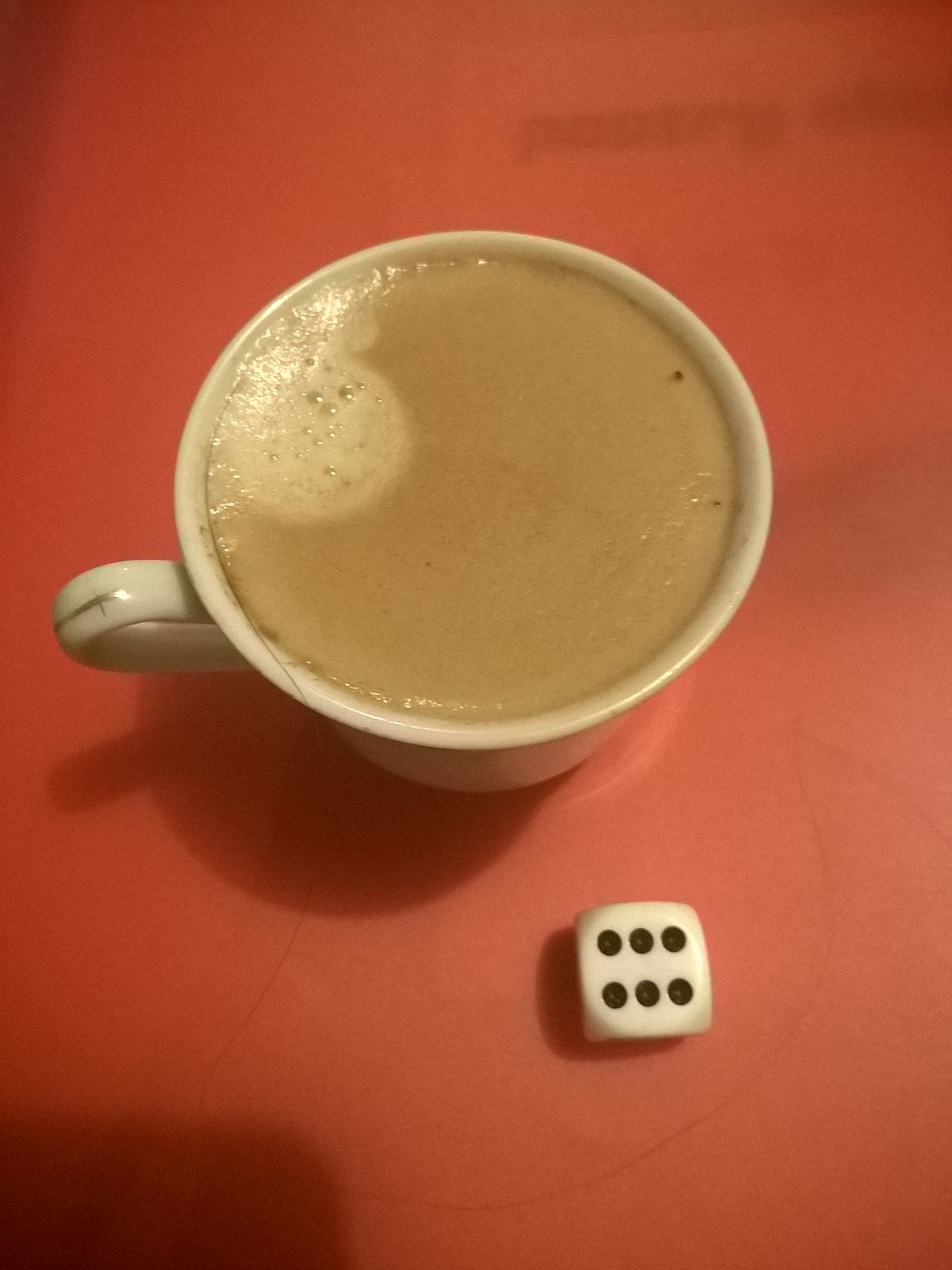The image showcases an off-white coffee cup resting on an orange table. The top of the handle features a thin gold strip, while a noticeable black hair is draped over the rim near the handle, extending down and curving around to vanish off the right edge of the picture. The cup is filled with a medium brown beverage, most likely coffee, topped with foam and bubbles on the left-hand side. Within the bend of the hair, a six-sided die is visible on the table, showing the number six. The die is also off-white with black pips. There is a subtle shadow in the corner that hints at a rectangular object reflecting a piece of paper with the word "Poetry" on it.